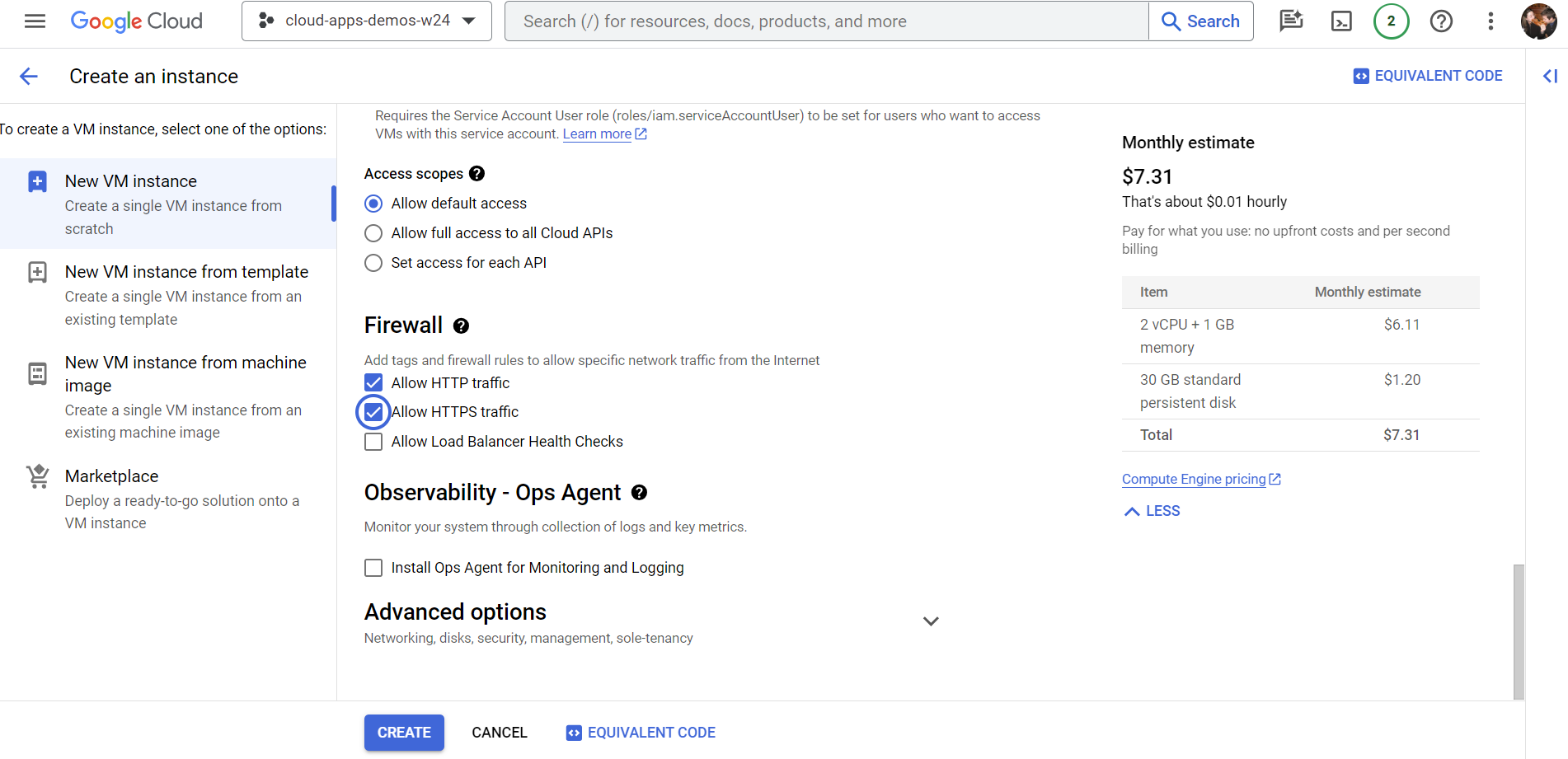**Detailed Caption for the Image:**

The image depicts a screenshot of a Google Cloud Platform (GCP) interface with a predominantly white background. At the top of the page, the Google logo is prominently displayed on the left, followed by the word "Cloud" and a search bar. Below this navigation bar, the page title "Create an Instance" is accompanied by a blue arrow pointing to the left.

The main content is organized into three vertical columns:

1. **Left Column: VM Instance Options**
   - It provides instruction: "To create a VM instance, select one of these options."
   - The options listed are:
     - New VM instance
     - New VM instance from template
     - New VM instance from machine image
     - Marketplace

2. **Middle Column: Configuration Settings**
   - It explains the requirement: "Requires a service account user role (roles/IAM-serviceAccountUser) to be set for users who want to access VMs with this service account," followed by a hyperlink labeled "Learn more."
   - Below this, settings for access scopes are shown:
     - "Allow default access" (selected)
     - "Allow full access to all Cloud APIs"
     - "Set access for each API"
   - Firewall options:
     - "Add tags and firewall rules to allow specific network traffic from the internet," with:
       - "Allow HTTP traffic" (selected)
       - "Allow HTTPS traffic" (selected and circled)
       - "Allow load balancer health checks"
   - Observability ops agent:
     - "Monitor your system through collection of logs and key metrics."
     - Option to "Install ops agent for monitoring and logging advanced options."

3. **Right Column: Cost Estimate**
   - Displays a cost estimate for the VM instance:
     - "Monthly estimate: $7.31 (approximately $0.01 hourly)"
     - Highlights: "Pay for what you use, no upfront costs, and per-second billing."

At the bottom of the screenshot, three action buttons are visible: "Create," "Cancel," and "Equivalent code."

This detailed organization provides a comprehensive overview of the VM creation process on Google Cloud Platform, including options, requirements, and estimated costs.